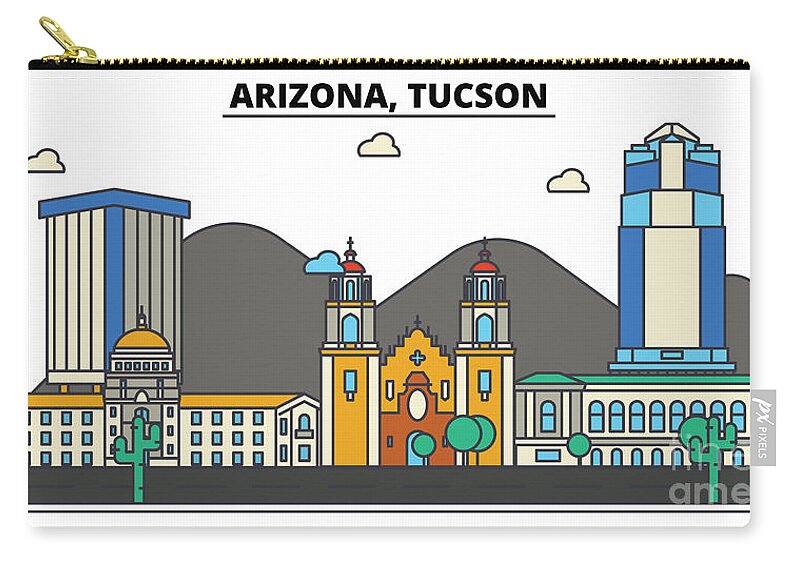The image depicts a small white pouch with a gold zipper at the top, complemented by a black strip. The text "Arizona Tucson" in all capital letters and a sans serif font is prominently displayed at the top, underlined in black. The design features a colorful graphic representation of Tucson's skyline, set against gray mountains. Central to the skyline is a church building with a cross and a yellow front. To the left is a dome-shaped building, edged in blue, and to the right is a tall, blue building. There are several cacti in the foreground, indicative of the Sonoran Desert. The composition includes a variety of colors—orange, yellow, green, blue, light blue, beige, white, and black—adding vibrancy to the scene.